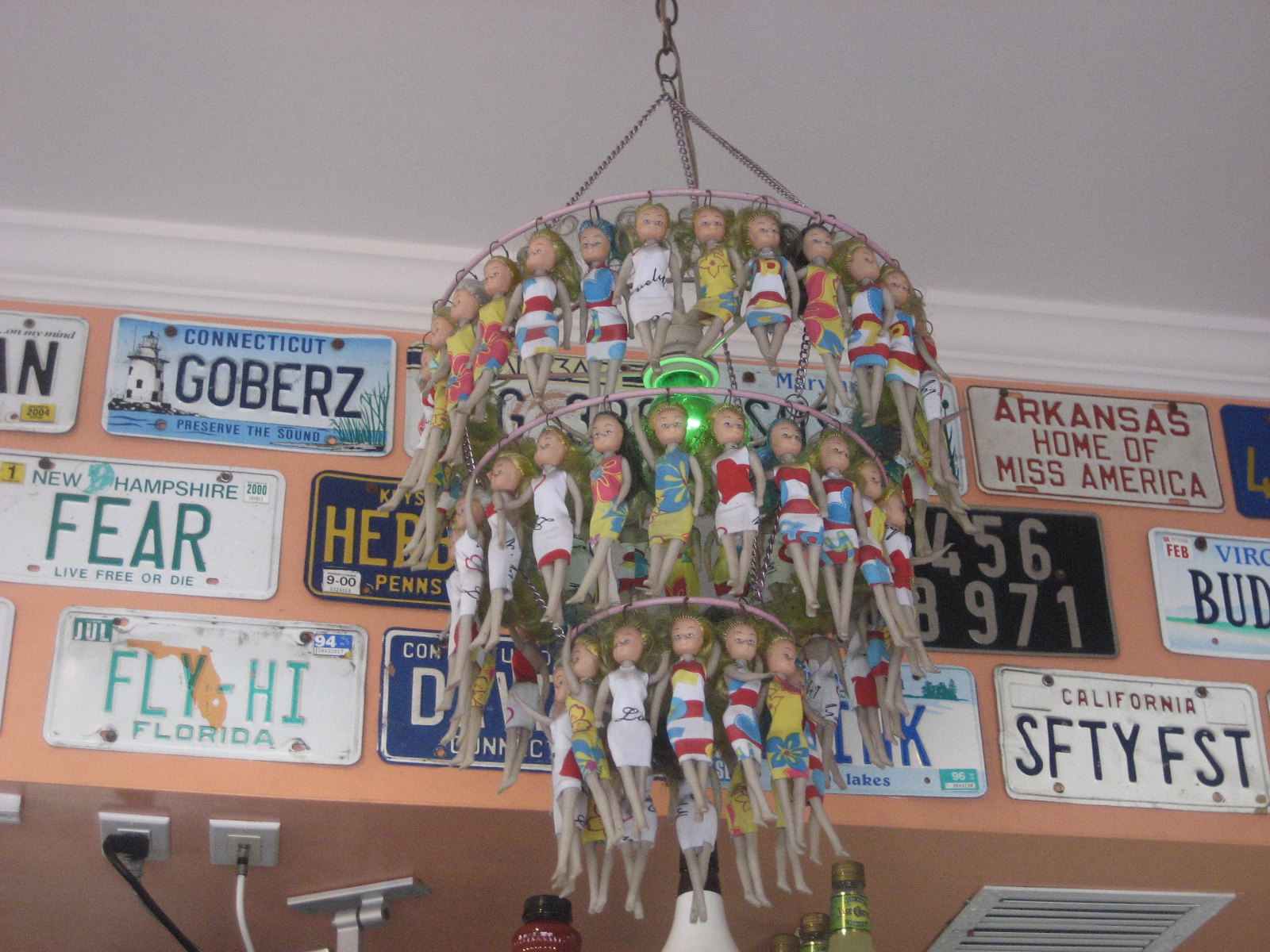The indoor setting features a unique and eclectic décor, highlighted by a white ceiling. Just below the ceiling, where the wall comes down in pink or orange hues, there is a striking display of novelty license plates from various states including Connecticut, New Hampshire, and Florida. These plates notably carry playful slogans like "Go Birds," "Fear," and "Fly High," rather than their standard state names. 

Dominating the center of the image is the main subject: an unusual chandelier crafted from Barbie dolls, each suspended by their hair. The chandelier is embellished with red wire and features a green light bulb at its core, casting an eerie yet fascinating glow. Surrounding this focal point, the wall space transitions into a collection of variously colored license plates, including others from California, Virginia, and Arkansas, while some plates are partially obscured. Additional details include a vent located in the bottom right and some electrical plugs in the bottom left, contributing to the overall quirky and vibrant atmosphere of what appears to be a personalized space, potentially a bedroom or man cave. The color palette of the image is diverse, incorporating shades of white, gray, silver, green, light blue, yellow, orange, blue, black, red, pink, and purple.